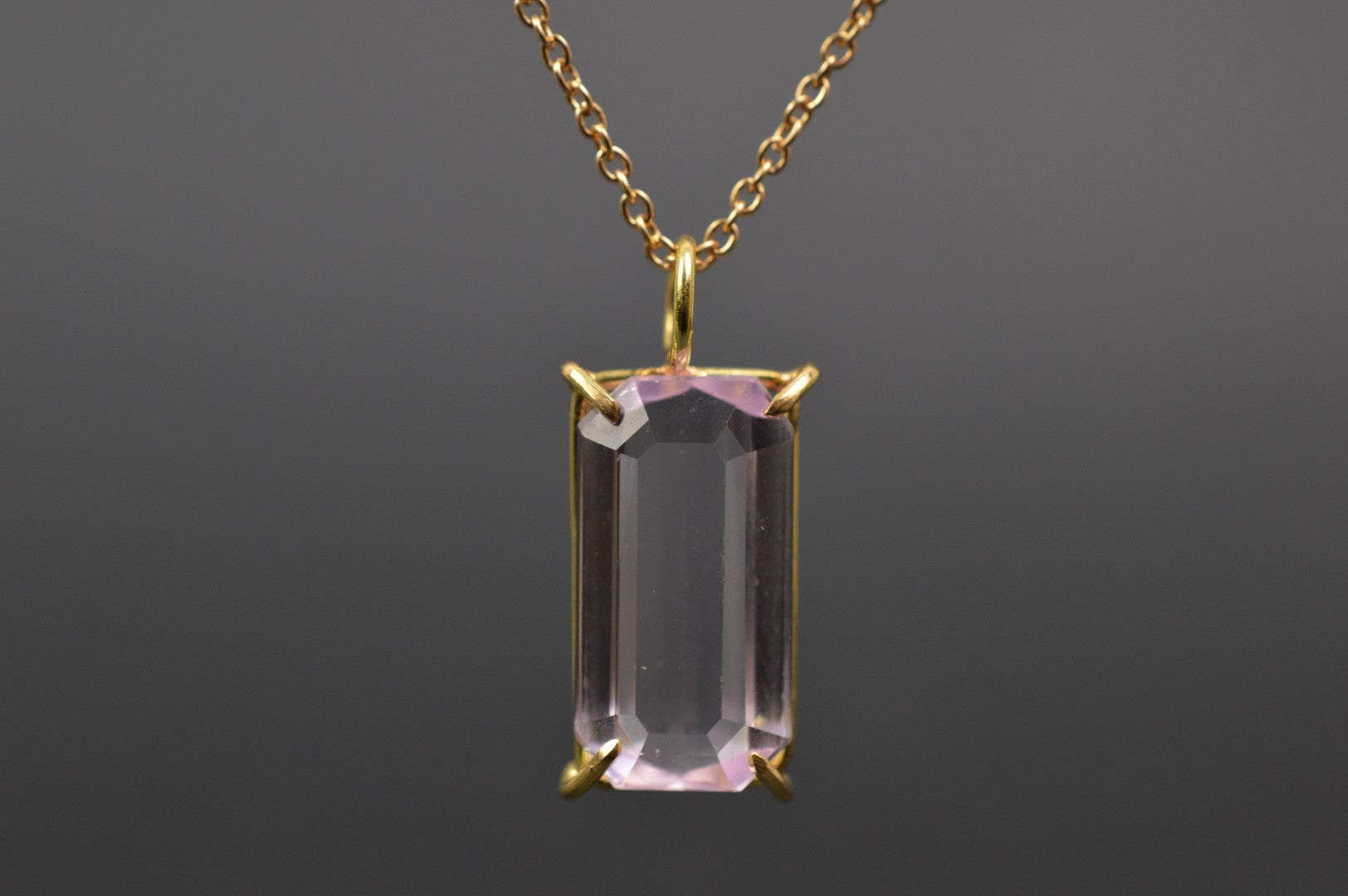A gold-linked necklace with a rectangular, emerald-cut purple gemstone pendant is positioned centrally over a gradient gray background that transitions from lighter gray at the top to darker gray at the bottom. The gemstone, possibly an amethyst or rosy quartz, measures about an inch in length and a quarter-inch in width. It is housed in a shiny gold setting and secured by four gold prongs. At the top of the setting is a gold ring, partially obscured, through which the gold chain loops. The necklace and pendant appear to have a slightly worn finish, suggesting they may be preloved or vintage.